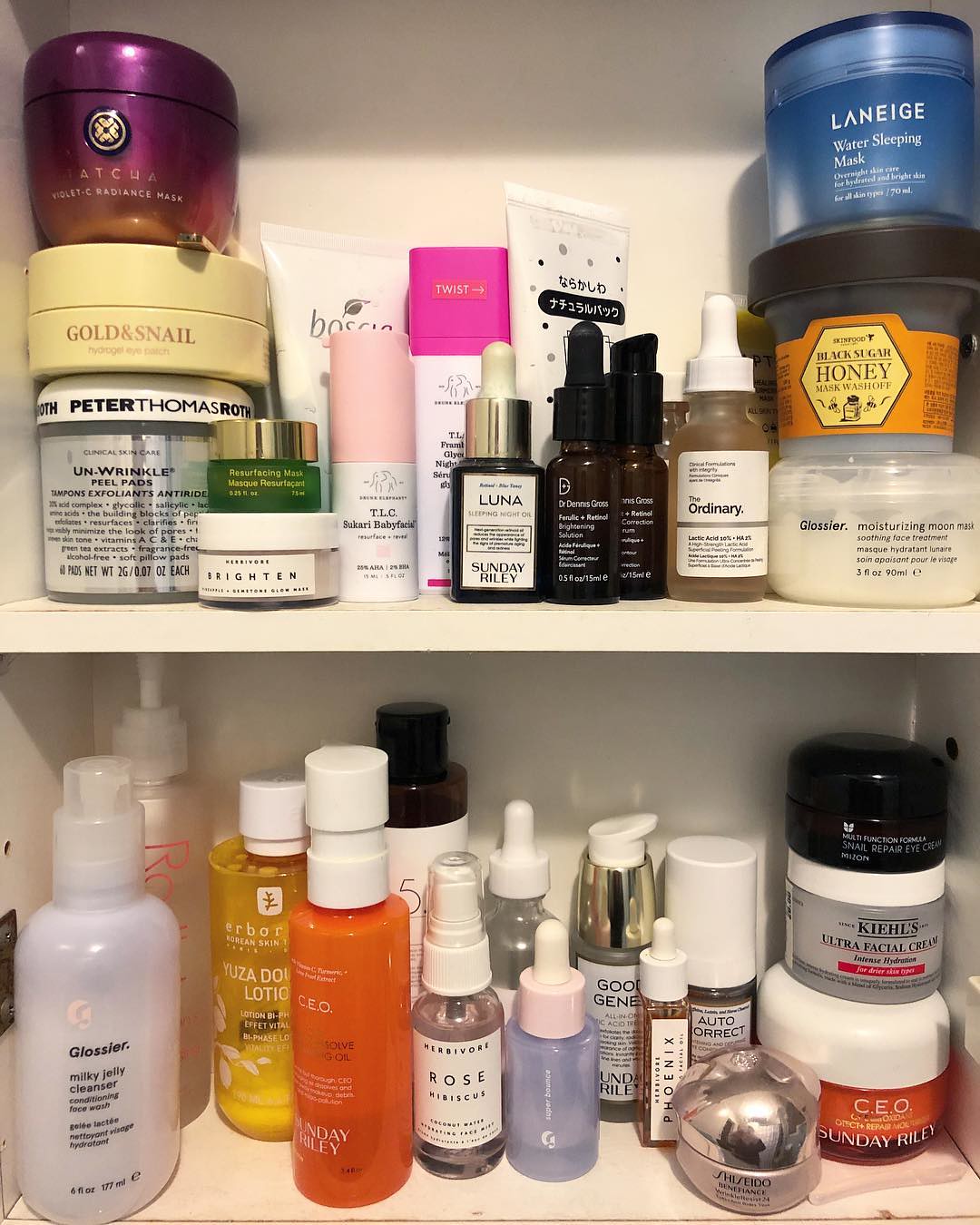A neatly organized two-shelf dresser serves as a dedicated storage space for an assortment of high-end skincare products. The top shelf displays a variety of prestigious brands such as Tatcha, Peter Thomas Roth, Basha, Tata Harper, Drunk Elephant, Laneige, The Ordinary, and Dr. Dennis Gross, alongside a couple of items from Glossier. This shelf showcases three moisturizers stacked on top of each other on both the left and right sides, while the center features single, upright bottles. 

The bottom shelf continues the trend of luxury skincare with additional items from the same brands, including highly popular products like Good Genes and C.E.O. Moisturizer by Sunday Riley. In the right corner of the bottom shelf, another trio of moisturizers is stacked, contributing to the organized yet abundant display. Products in various shapes, particularly round jars or tubs, are skillfully stacked to maximize the space and maintain an orderly appearance.